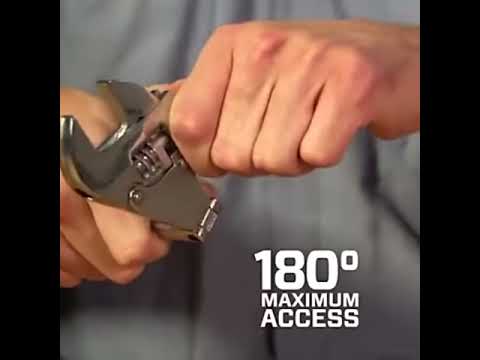The image is a close-up of two hands demonstrating the use of a metal tool, most likely a pair of pliers or a similarly adjustable wrench, focusing on its capability to bend at odd angles. The individual, identified by their Caucasian skin tone and wearing a gray shirt, uses their right hand to firmly grasp the tool while the left hand adjusts the dials to open or close it. The background features a gray, tapestry-like material that resembles a window curtain, providing a slightly blurry backdrop that emphasizes the hands and tool in the foreground. The image is bordered on both sides with black outlines, and in the lower right-hand corner, white text reads "180 degrees maximum access," highlighting the tool's operational range. Shadows of the hands are visible against the gray background, enhancing the depth and focus on the demonstration.